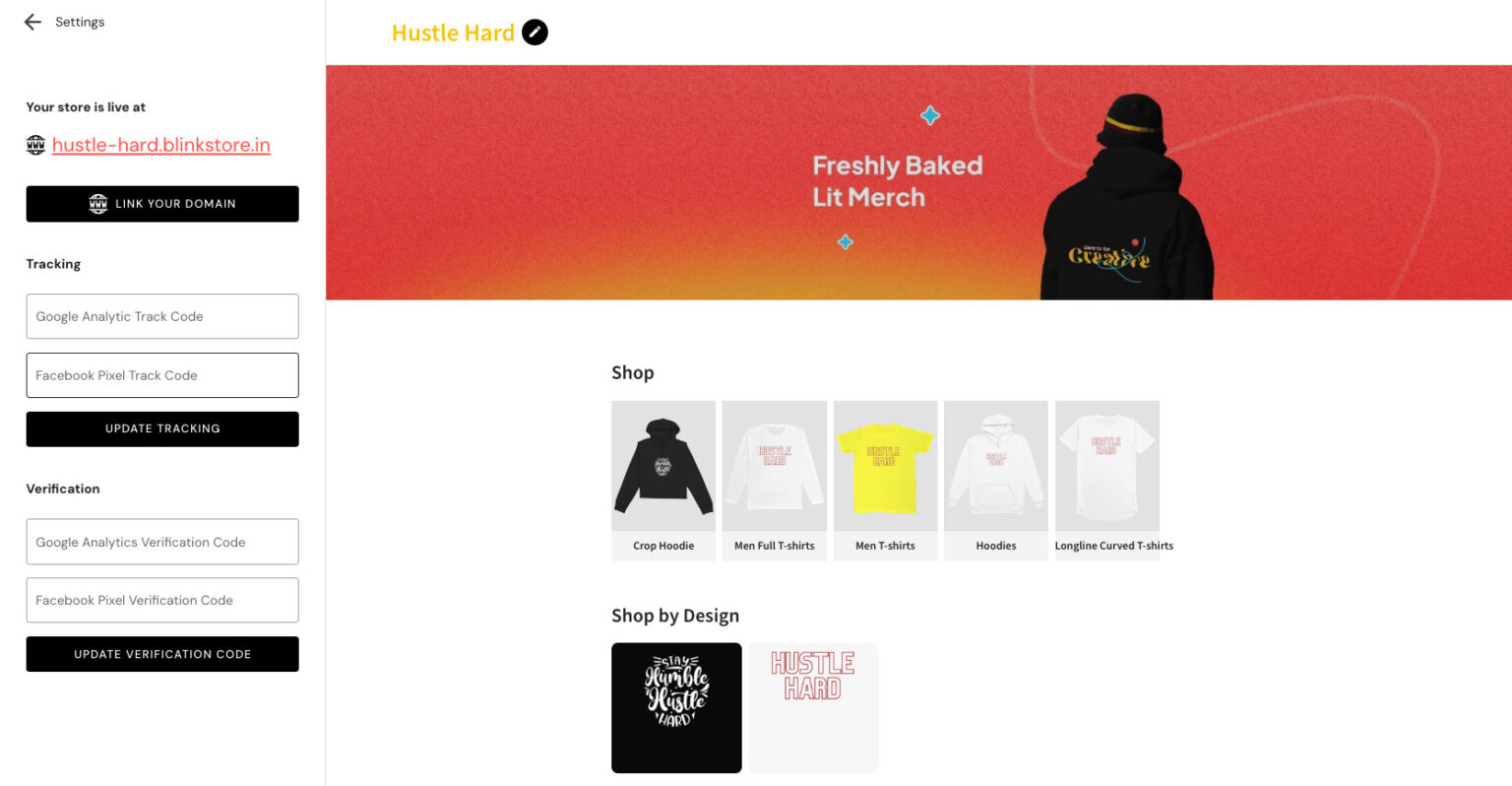This image showcases a website interface for an online store with the URL "hustledashhard.blinkstore.in." On the right side of the webpage, a strikingly vivid rectangular banner features the text "Freshly Baked Lit Merch" in bold characters. This banner starts with a deep red color at the top, transitioning smoothly to a bright orange at the bottom. 

Dominating this rectangular space is a graphic that notably resembles a figure wearing a sweatshirt emblazoned with the word "Creative" along with a hat; although the figure itself isn't fully visible, the design suggests a stylish and modern vibe. Adding to the dynamic layout, a sleek white swoosh line elegantly cuts through this area. 

On the shopping section of the website, users can browse a variety of apparel, including crop hoodies, men's full t-shirts, hoodies, and longline curved t-shirts. The store also emphasizes its unique designs, spotlighting inspirational slogans such as "Stay Humble, Hustle Hard" and "Hustle Hard."